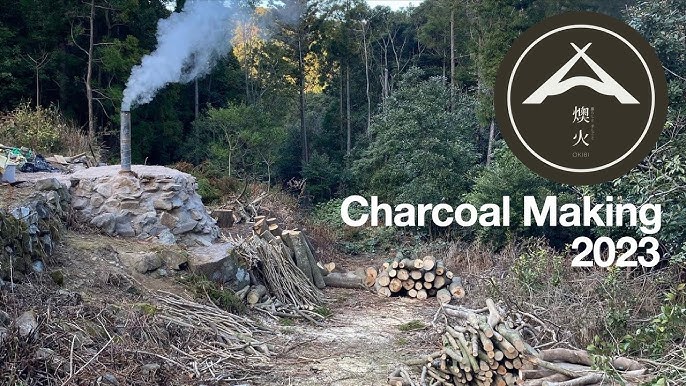This image captures a dry, wooded outdoor area featuring a mix of thin, green trees emerging from gray trunks, alongside a large green bush. Scattered throughout are tan and white sticks protruding from the ground, giving the scene a distinctly arid feel. Towards the bottom of the photo, cut logs are neatly stacked, possibly along a small, cleared pathway. On the left side of the image, a man-made stone structure is visible, with a metal pole extending from it, emitting white smoke. Above the pole and smoke, there is a brown and white symbol in a circular logo, with the text "Charcoal Making 2023" written in white.